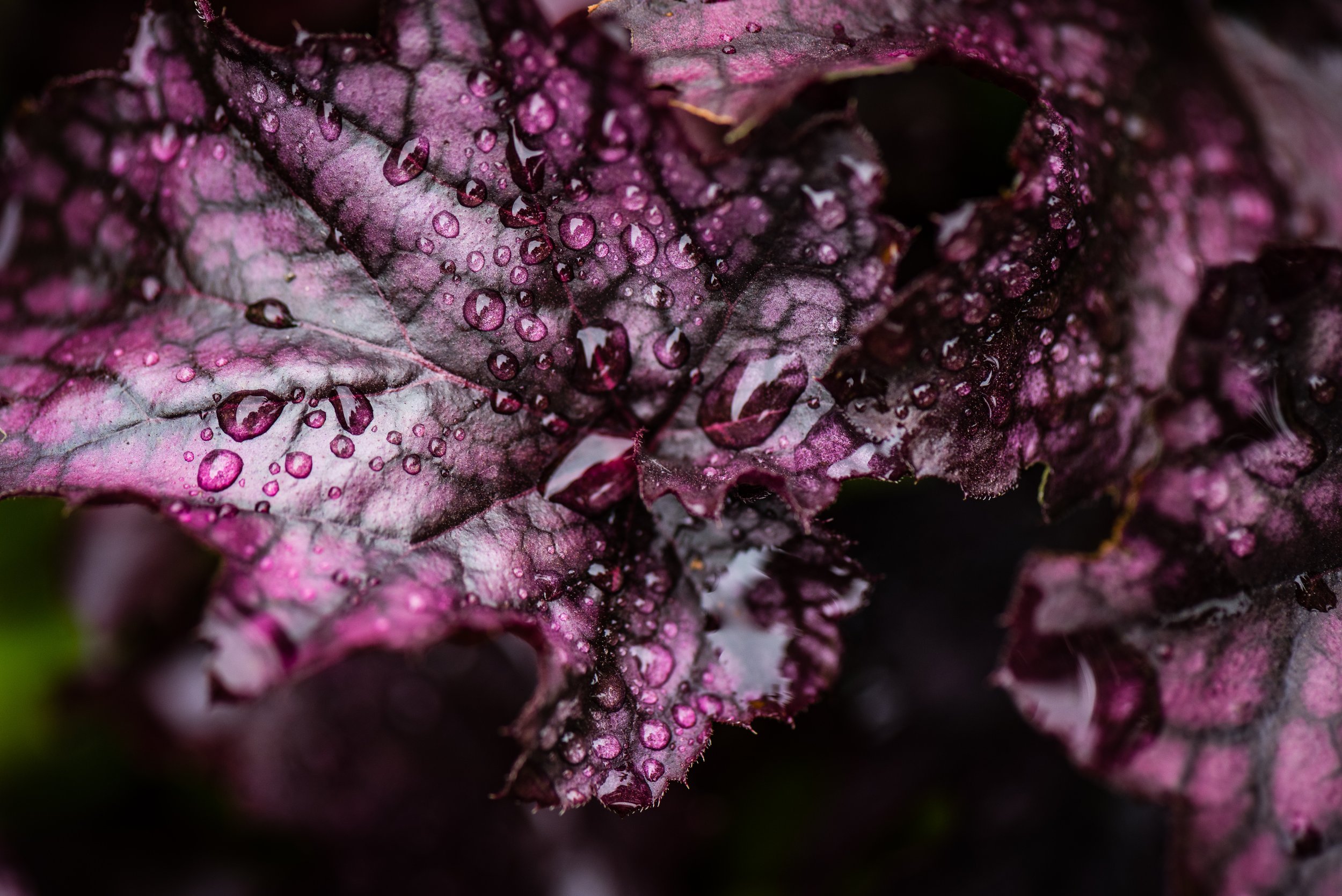The image captures a detailed close-up of a striking purple-colored leaf adorned with prominent dark black veins. Water droplets delicately scattered across the leaf's surface reflect various colors, suggesting a recent rainfall. The background is bathed in shadowy darkness, contrasting sharply with the vibrantly illuminated leaf. Multiple leaves, both left and right, share this vivid coloration, providing a cohesive visual theme. A noticeable patch of green vegetation peeks out from the bottom left corner, adding a touch of natural diversity to the scene. Though no stem is visible, the overhead lighting from a presumably overcast sky highlights the clarity and intricate details of the leaves, emphasizing the high surface tension of the water droplets that remain unabsorbed.